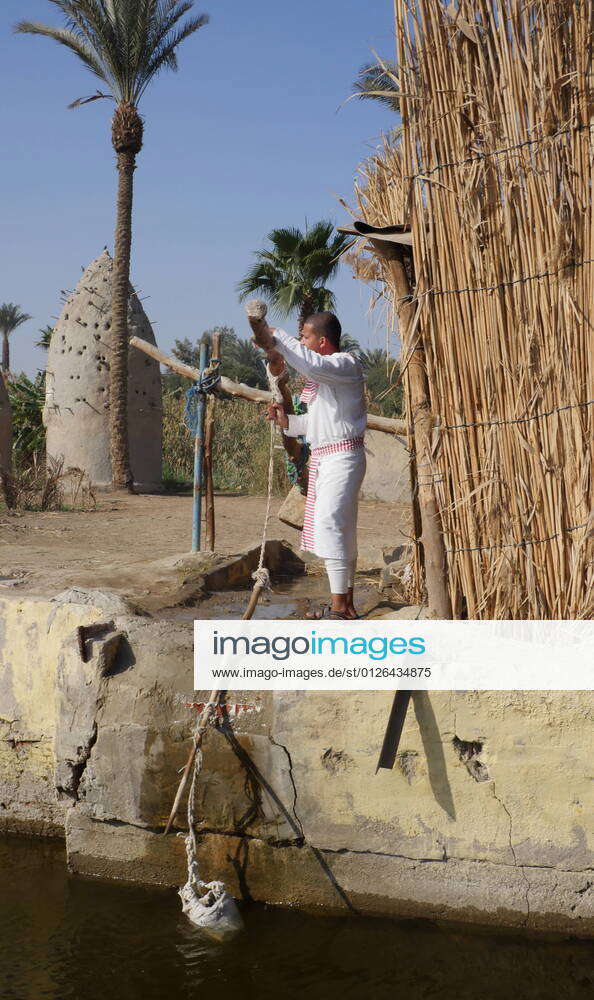The photograph depicts a man dressed in a white shirt, white pants, and sandals, standing by a dusty, riverbank beside a small cliff. The water at the bottom portion of the image appears reddish-brown and murky. The man is engaged with a contraption consisting of a thick, tree-like pole with a blue rope around it. This pole is perpendicular to another pole behind him and has a further rope extending towards the viewer, then descending over the cliff edge. He seems to be dipping or pulling a bag from the water. 

To the man's right is a large, sturdy wall made of straw-like plant material, reinforced with little ropes. This structure is supported by a thinner log at its corner. The background features a blue sky, some bushes, and a palm tree. Additionally, there is a cylindrical structure with a sharp roof resembling a bullet. Near the man's feet is a white rectangle containing the text "Imago images" with "Imago" in black and "images" in blue, followed by a website URL.